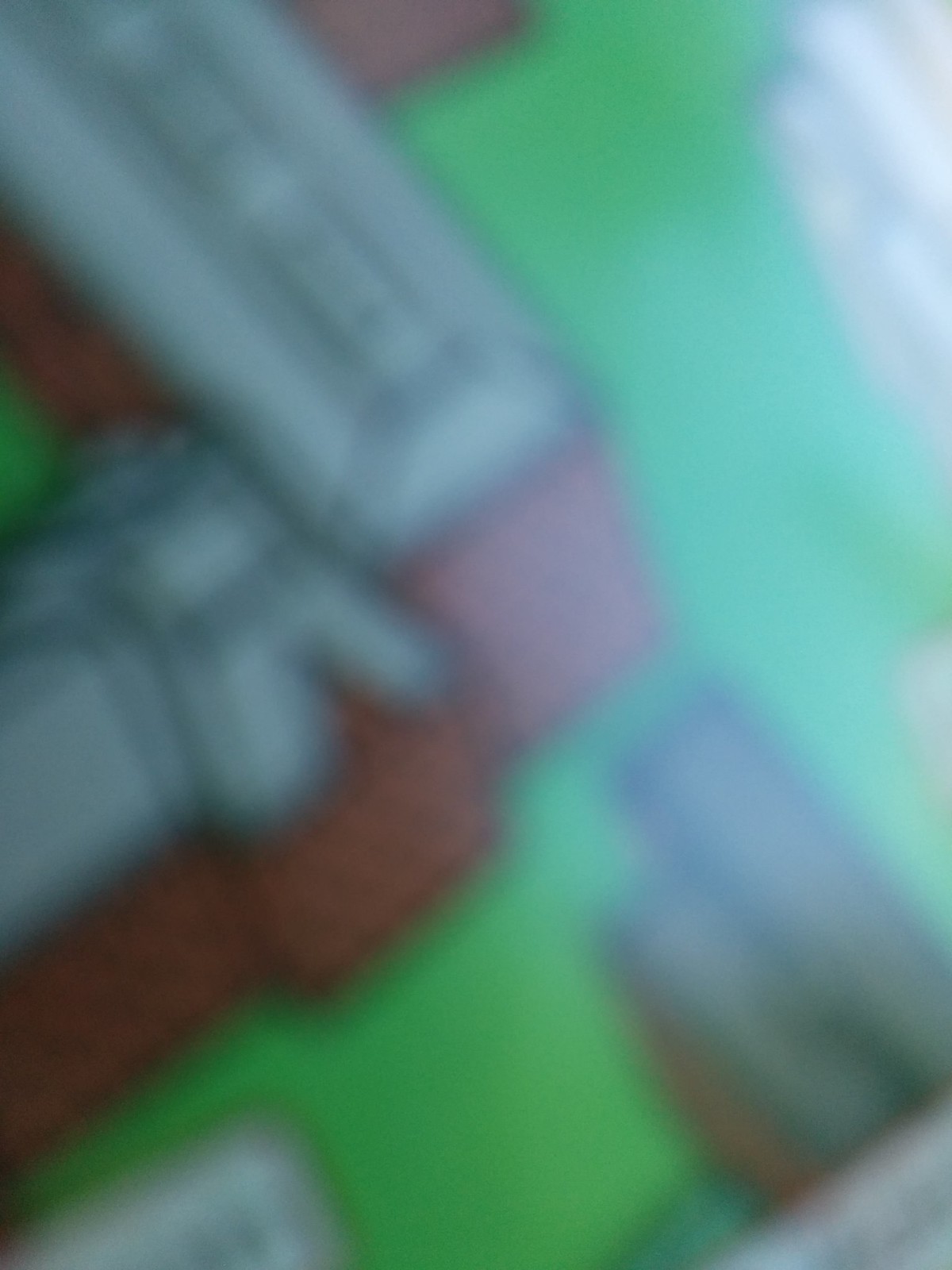The image is highly blurred, making it difficult to discern specific details. The predominant colors appear to be in a lime to mint green palette, accompanied by accents of brown, white, and black outlines. There seems to be a light source producing a white sheen, further contributing to the lack of focus. Despite the blurriness, the image features symmetrical shapes, including rectangular forms and potentially square elements. One focal point in the bottom right corner resembles a vertical building, akin to a cityscape. It is surmised that this is an illustration or a painting, rather than a photograph or a real-life scene. Some speculate that it could be a mural or decorative piece, perhaps resembling a child's rug depicting buildings and roads.